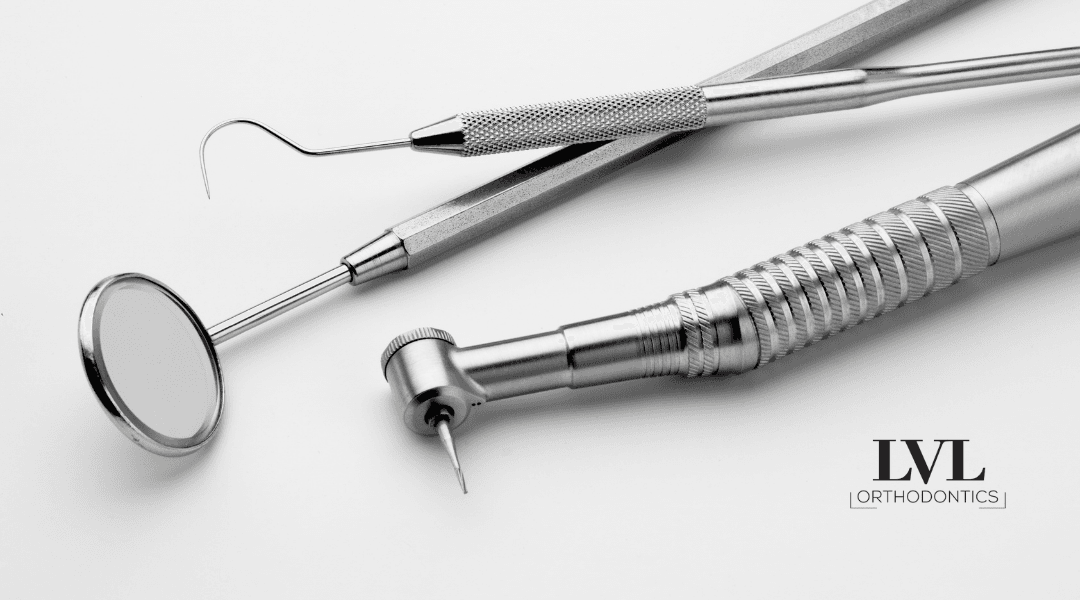This black and white photograph, captured in landscape orientation, showcases three orthodontic tools against a clean white background. The rectangular image is proportioned with its top and bottom sides twice as long as its left and right sides. In an almost horizontal configuration, the sleek stainless steel instruments converge from the top right corner, extending across nearly the full width of the image before their handles exit the frame. 

At the forefront, a stainless steel needle attached to a thick tube resembles a drill, pointing towards the bottom center of the image. Slightly overlapping with the needle tool, a reflective mirror with a circular face and smooth handle lies beneath a textured, pointed metal hook tool. Both the mirror's frame and the hook's handle share the same chrome material, creating a harmonious visual texture.

In the bottom right corner, the bold black text "LVL" stands above smaller, finely detailed black text that reads "orthodontics," providing a clear identifier for the brand. This photograph perfectly captures the polished precision of the dental instruments, emphasizing their streamlined forms and the professionalism of the orthodontic practice.